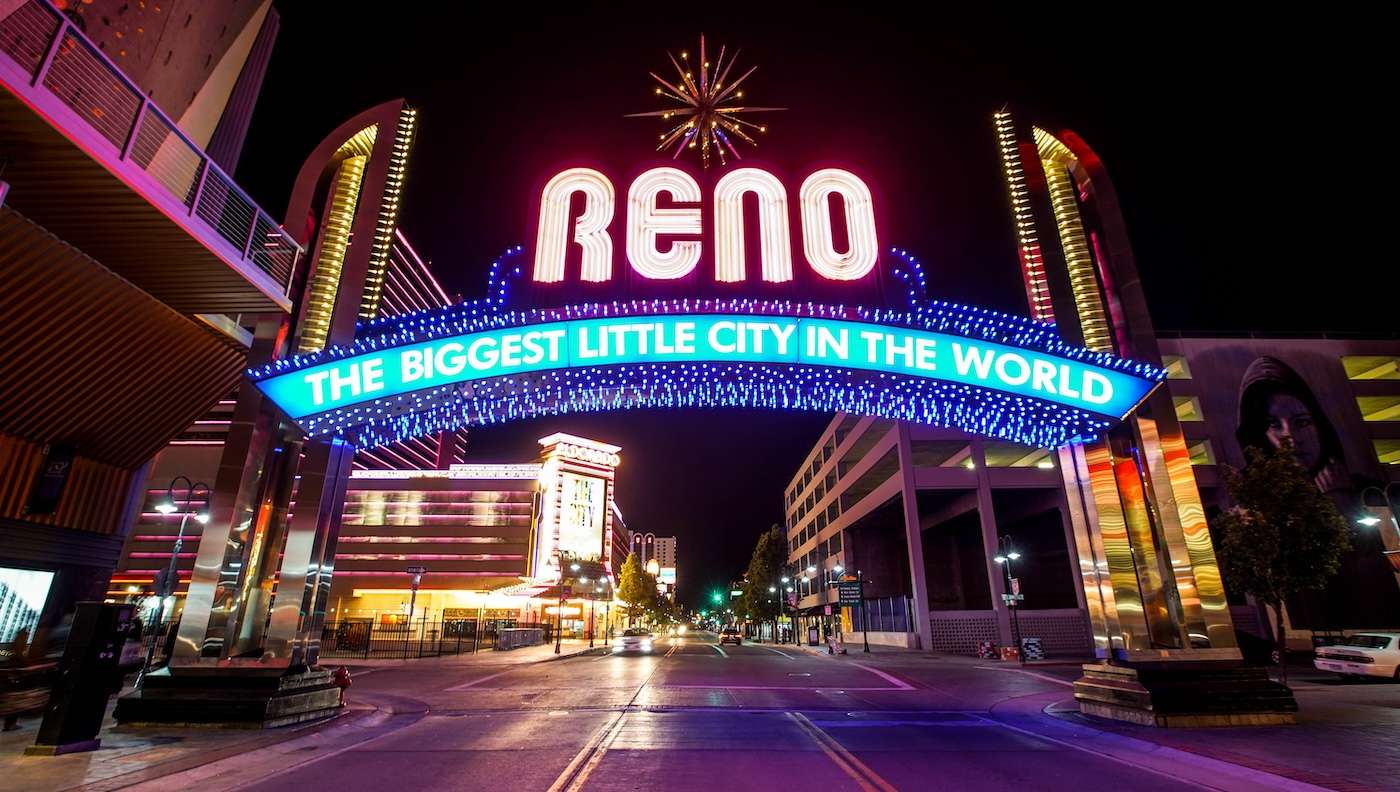This nighttime photograph captures the vibrant entrance to Reno, Nevada, famously known as "The Biggest Little City in the World." The image is taken from the middle of the road, offering a driver's perspective. Dominating the scene is a large, eye-catching archway spanning the street, with "Reno" illuminated in prominent white neon lights. Directly below, a blue banner with white lettering declares the city's moniker. This iconic sign is supported by two substantial Art Deco-style posts on either side of the street.

Beyond the arch and slightly to the left, the El Dorado shopping center or casino glows with its name in large white neon letters, enhancing the scene's lively ambiance. The street, flanked by buildings reminiscent of Las Vegas casinos, appears to be lightly trafficked with several cars heading towards the foreground, their headlights piercing the night. Streetlights, which stretch into the distance, cast a green hue on the crossroad further emphasizing the city's clean and orderly appearance. The Reno sign itself radiates a mix of dark purples and blues, contributing to the festive, casino-like atmosphere that characterizes this 'mini Las Vegas.'